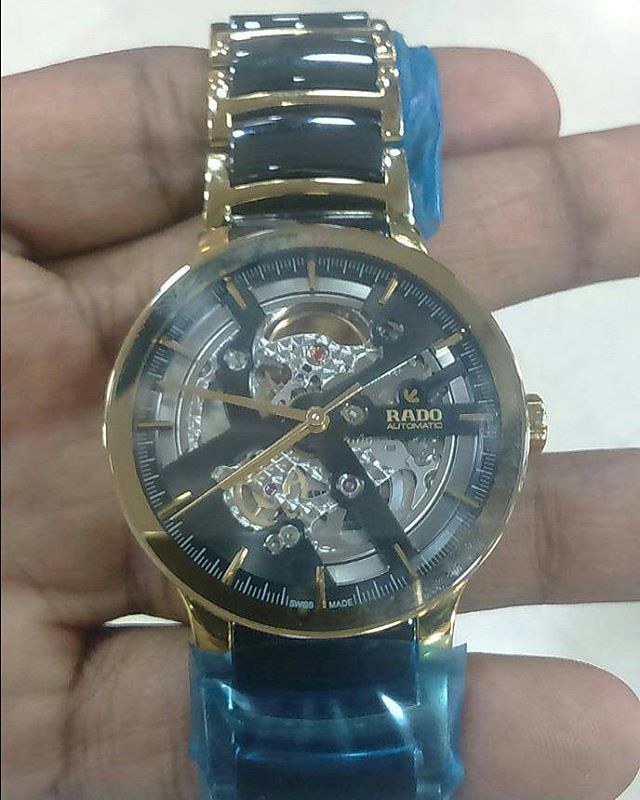In this image, set against a very light blue background, a man's hand is prominently featured, showcasing a remarkably unique watch. The watch features an intricately designed strap with dark blue panels complemented by elegant gold trims and light blue accents. The watch's gold exterior housing frames a sophisticated black face, with the brand name "RATO" emblazoned in gold letters alongside the word "automatic." The translucent black face subtly reveals the intricate inner workings of the timepiece, adding a touch of mechanical allure. Completing the luxurious design, the watch boasts sleek gold hands, emphasizing both its functional and aesthetic appeal.